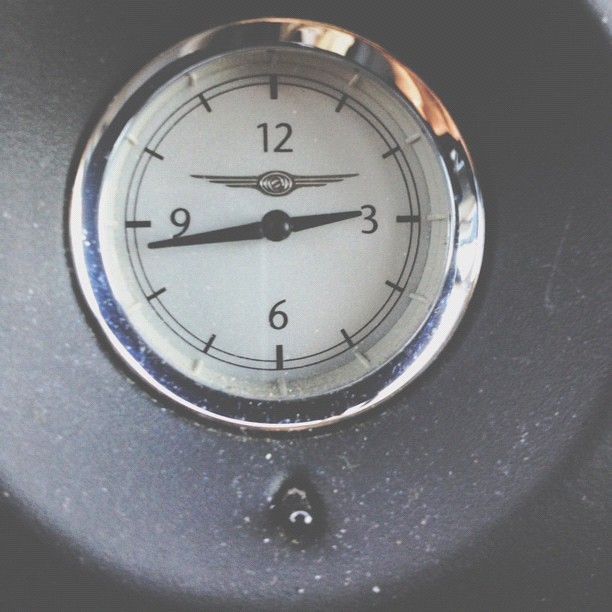This image features a miniature clock embedded within a sleek, black casing, which appears to be made of plastic or a similar material. The clock face is simplistic, presenting only the numbers 12, 3, 6, and 9, with small dashes marking the other hours. The clock face also bears a logo reminiscent of automotive emblems, potentially suggestive of a luxurious or high-end brand. The resemblance to a car badge, along with the compact design, indicates that this clock might be an integral part of a vehicle's dashboard or interior accessory. The overall detail is minimal, likely due to the diminutive size of the timepiece.